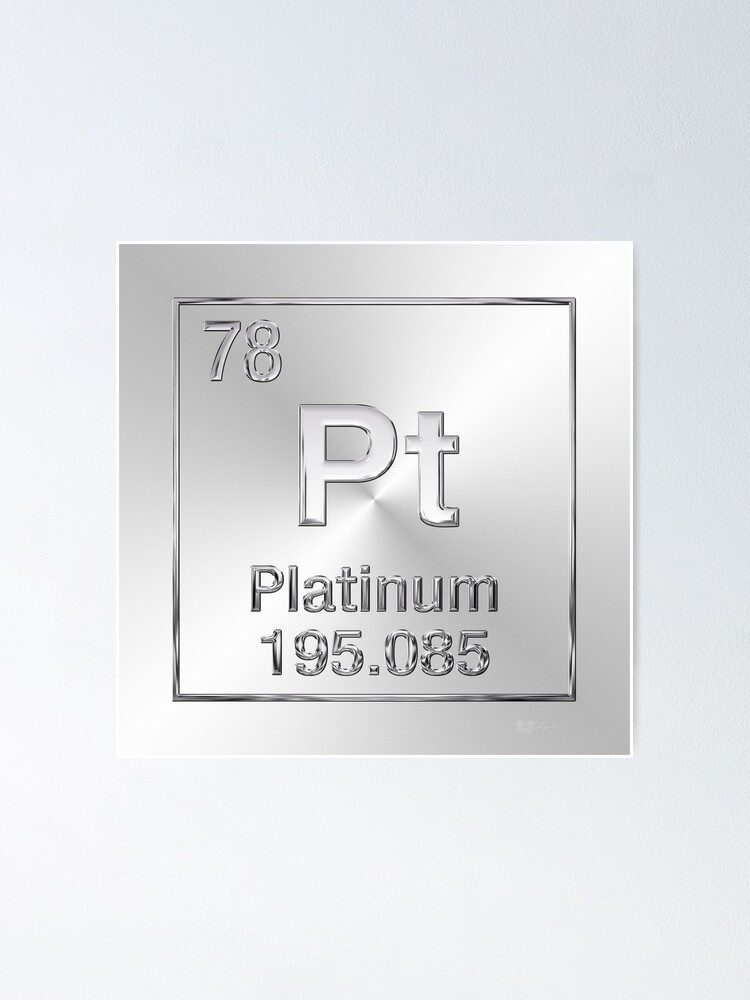This detailed descriptive caption combines and refines the input from all three sources:

This is a close-up photograph of a square metallic plaque representing the element platinum in an atomic element chart style. The plaque, set against a white background that fades to grey at the top right, features a shiny silver border and a slightly raised inner border of the same material, giving it a darker appearance. In the top left corner of the plaque is the atomic number 78. Centered within the plaque are the symbols Pt, with 'P' in uppercase and 't' in lowercase. Below the symbols, the word "Platinum" is inscribed in silver, followed by the atomic weight, 195.085. The entire image has a minimalistic and elegant presentation.